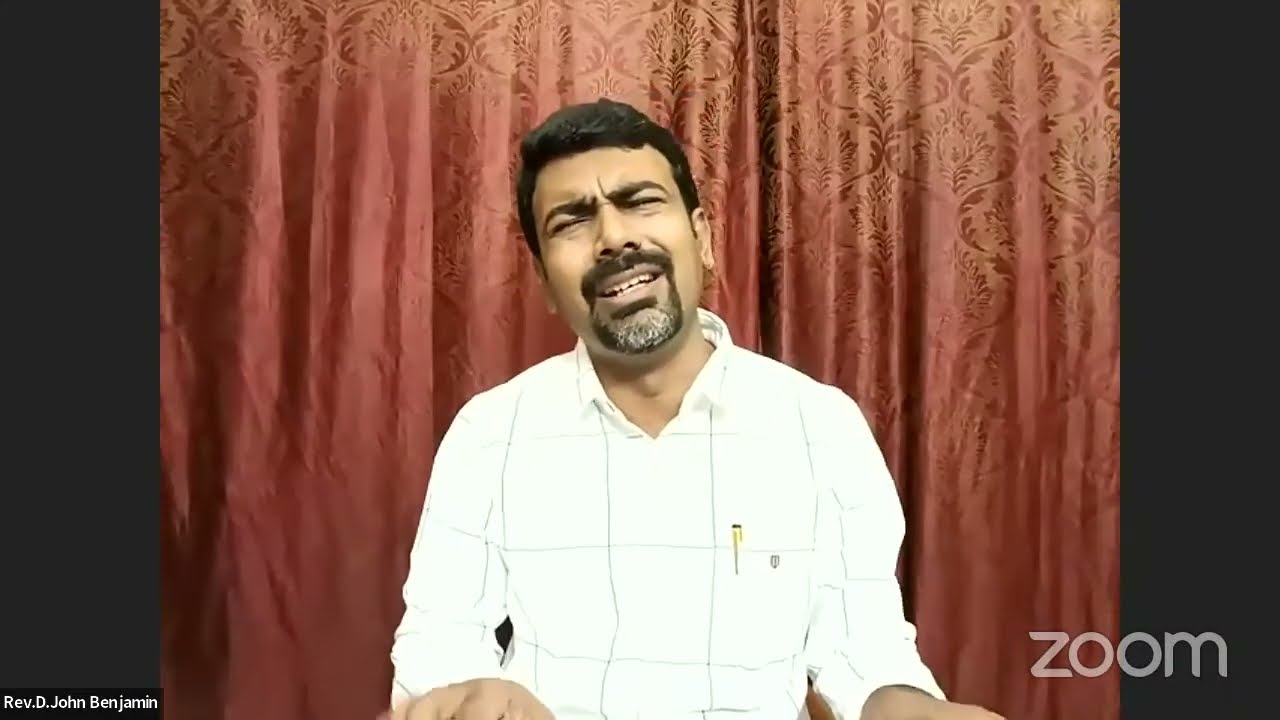The image depicts a middle-aged Indian man, positioned centrally and directly facing the camera, either standing or sitting. He is wearing a white button-down shirt with a grid pattern made up of widely spaced, thin gray stripes. The top button of his shirt is unbuttoned, and a gold pen is tucked into his chest pocket, which bears a small coat of arms symbol. The man appears to be in the midst of singing, with his forearms held parallel to the ground and each other, resembling a keyboard playing stance. Behind him, red curtains with a floral pattern form the backdrop, and while he seems to be participating in a Zoom call, a brand name "Zoom" is visible in the bottom right-hand corner. In the bottom left corner, the text reads "Rev. D. John Benjamin." The man’s expression is one of anguish or pain, adding a poignant intensity to the scene.